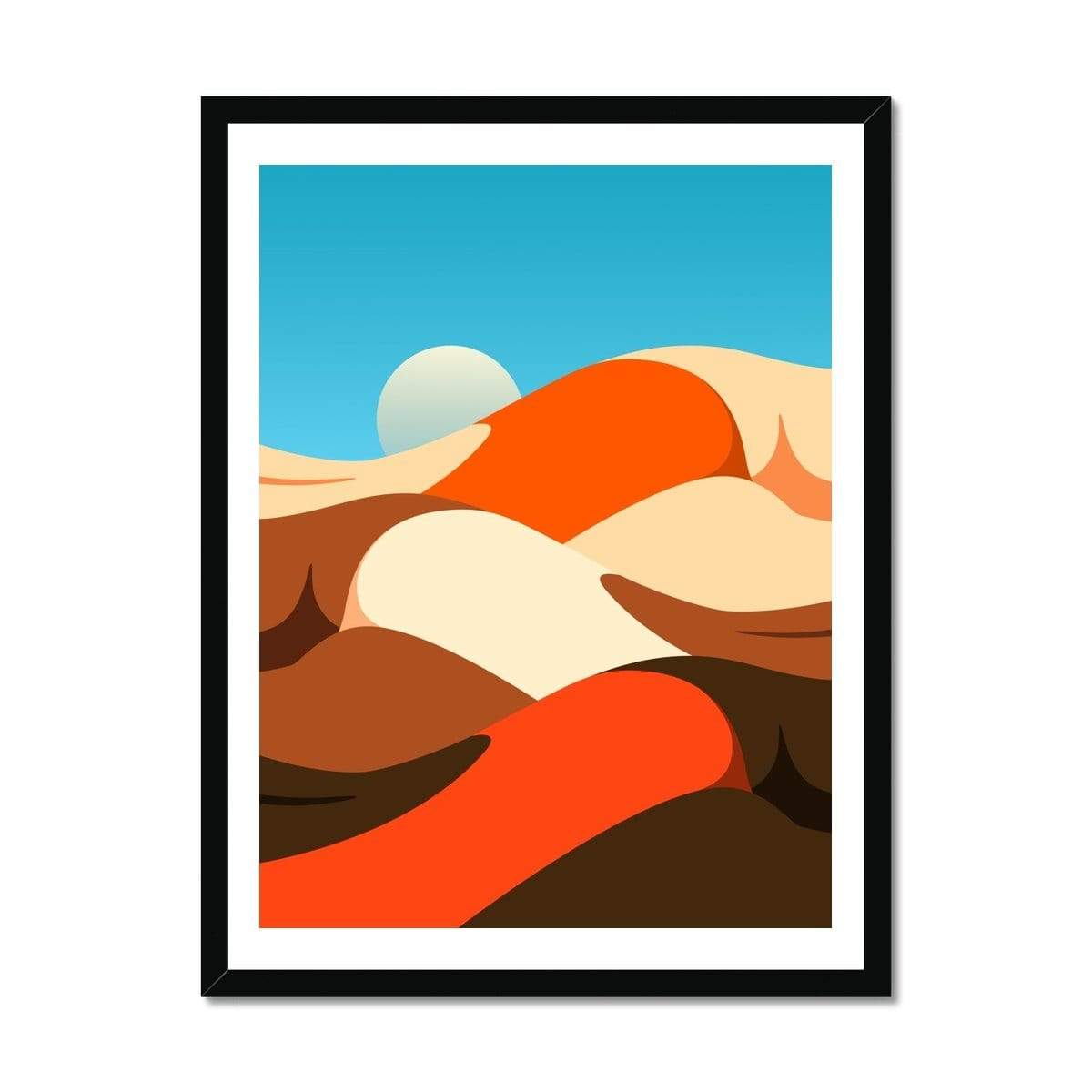The image is a framed wall art, centrally positioned against a white background. The artwork is encased in a black frame with a white border that accentuates the painting within. The artwork depicts an abstract landscape, likely computer-generated, featuring a desert theme with sand dunes. The dunes are rendered in various shades of beige, orange, and brown, forming smooth, heaped shapes that mimic a hill-like terrain. Over the horizon, a perfectly circular, white sun or moon rises, casting subtle shadows that hint at an outdoor setting. The sky above the dunes is a serene blue, completing the simple yet evocative outdoor scene. Despite its minimalist style, the image invites viewers to imagine different interpretations of its elements, from abstract shapes to more concrete landforms and celestial bodies.